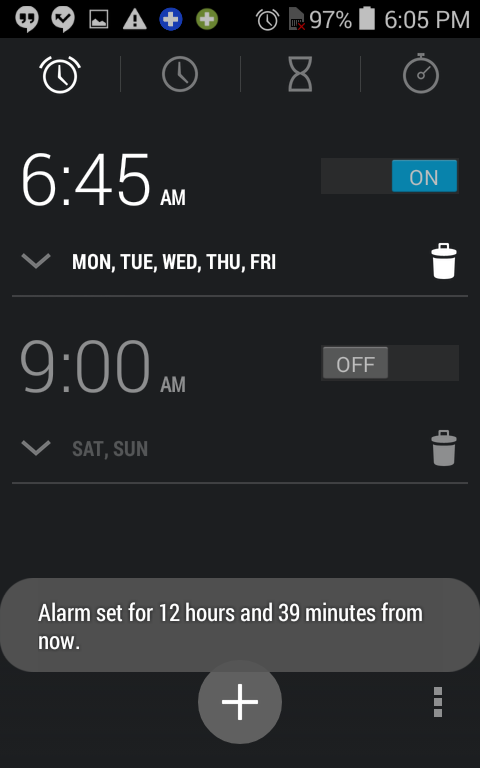The image depicts a detailed view of a cell phone screen containing various icons and notifications. On the left side, there are text message indicators next to a triangle with an exclamation point, signaling an issue or alert. Nearby are two circular icons, one blue and one green, both marked with plus signs, indicating the option to add something.

Displayed prominently is an alarm notification with several icons related to time management. These include a white clock with external lines, a grey clock, an hourglass, and a stopwatch, all in grey. The displayed time on the phone is 6:05 PM, with the battery at 97%.

The white clock icon indicates a recurring alarm set for 6:45 AM from Monday to Friday, currently active as denoted by a blue "on" button. Beside it is a white trash can icon, allowing users to delete this alarm. Below it, another alarm is shown, set for 9:00 AM on Saturday and Sunday, marked as off, with a corresponding trash can icon.

A grey and white notification bubble at the bottom states an alarm is set for 12 hours and 39 minutes from now. Additional icons include a white circle with a cross in the middle and three vertically-aligned dots in the bottom right corner.

The primary colors in the image are green, blue, red, white, grey, and black.